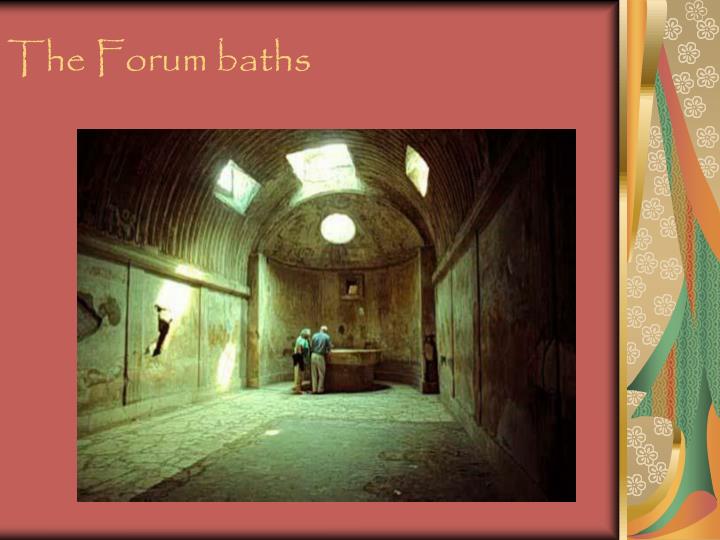This is a horizontal rectangular graphic showcasing an ancient archaeological site, titled "The Forum Baths" in yellow text at the upper left corner, set against a reddish-brown and orange backdrop. The main image inset within this graphic is a photograph of an ancient stone interior, possibly from Greece or Rome, featuring a dark, underground room resembling an apse of a church or a holy place, with a baptismal fount or bath. The room is dimly lit, with three skylights on the domed ceiling allowing sunlight to filter in. At the back of the room, there are two elderly individuals standing near what appears to be an altar or fountain. The walls are bare, with a beige-brown hue, enhancing the ancient ambiance. On the right side of the graphic is a multicolored floral and patterned section with gold, blue, and orange detailing, interspersed with white flowers. The inset photo is surrounded by a salmon-colored border, suggesting a web extraction, adding to the aesthetic depth of the overall presentation.